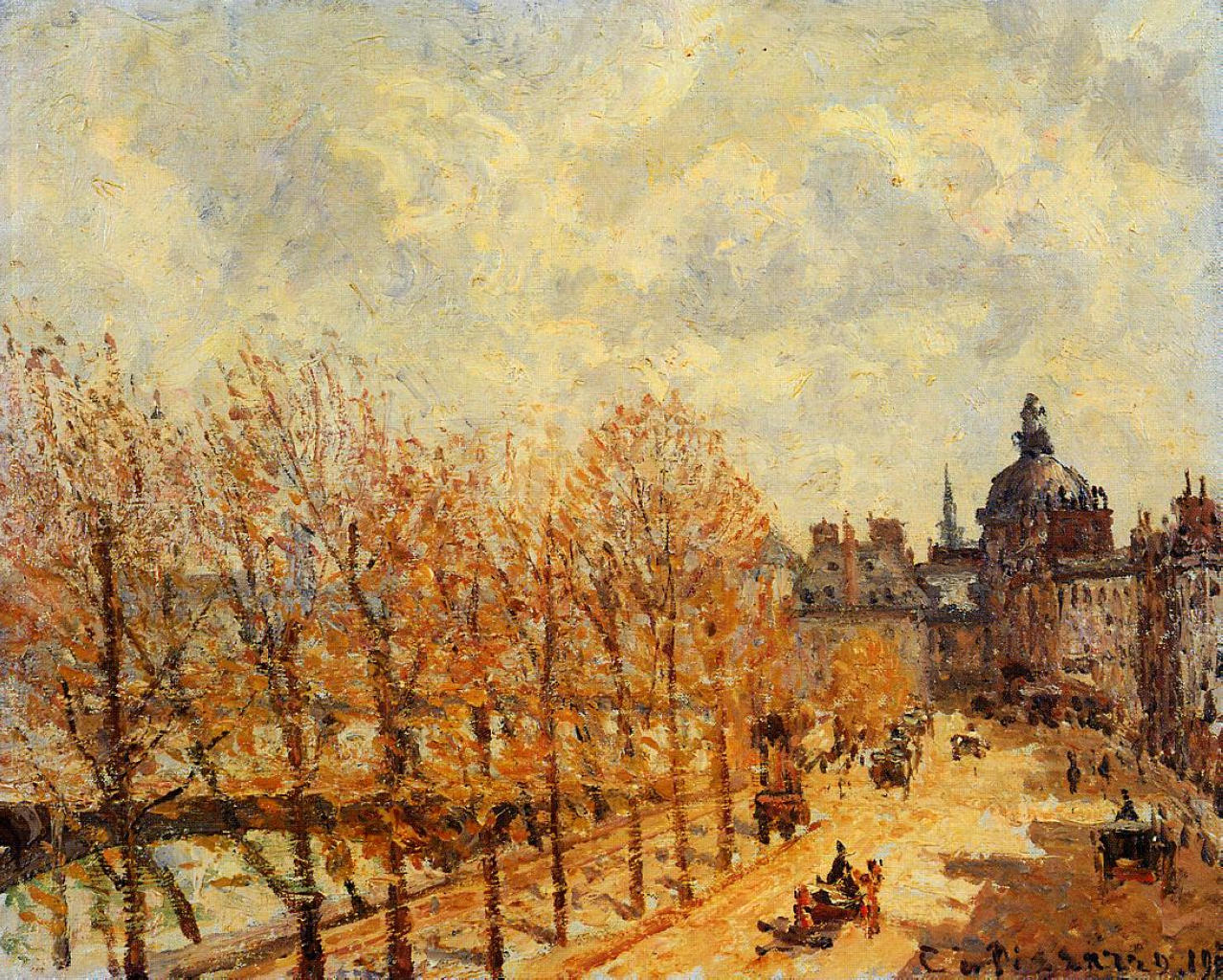This is an Impressionistic oil painting by French artist Camille Pissarro, depicting a lively scene of French town life in the 1800s. The view is from an elevated perspective, perhaps a rooftop, looking down on a bustling city street. On the left side, a stand of trees with orange and yellow leaves suggests the autumn season. Beyond the trees, there is a bridge and a body of water framed by a line of trees with brown trunks. Moving rightward, one can notice a woman sitting on a bench and several people walking along the sidewalk, wearing 1800s style dresses and costumes. Various modes of transportation, including horse-drawn carriages and buggies, populate the street, which appears light reddish-orange with a muddy brown section.

The cityscape in the background is rich with multi-story buildings predominantly colored in orange, yellow, and specks of maroon. The most prominent structures are a large basilica with a dome topped by a sharp spire in the center and a nearby church with a tall, thin spire. The sky above is filled with swirls of yellow, light green, gray clouds, and patches of blue. The signature "C. Pissarro, 18--" appears in black ink in the bottom right corner, marking the artist's handiwork. The overall atmosphere of the painting is vivid and dynamic, capturing the essence of a vibrant city during the daytime.